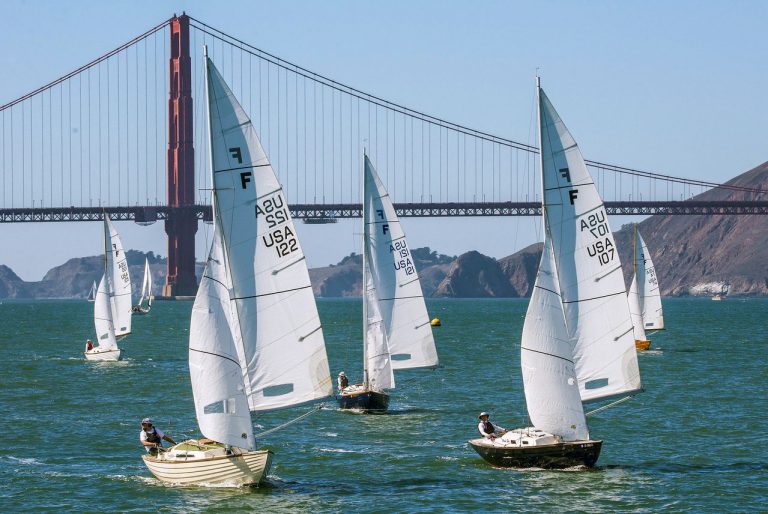The image captures a lively sailboat race taking place on a greenish-gray ocean, with a clear blue sky overhead. In the background, a mountain range stretches horizontally across the image, culminating in higher peaks on the right. A long suspension bridge spans the scene, its multiple cables connecting the structure to the supporting towers above. In the foreground and middle ground, there are six to seven sailboats with white sails, each featuring different alphanumeric texts and numbers, such as "ASU122 USA" and similar variations. The sailboats come in black, white, and brown hull colors. Single individuals are seen operating these boats, hinting at an organized competition. The predominant colors in the image are shades of blue, gray, and brown, which are reflected in the sky, ocean, mountains, bridge, and the boats, creating a harmonious and dynamic composition.